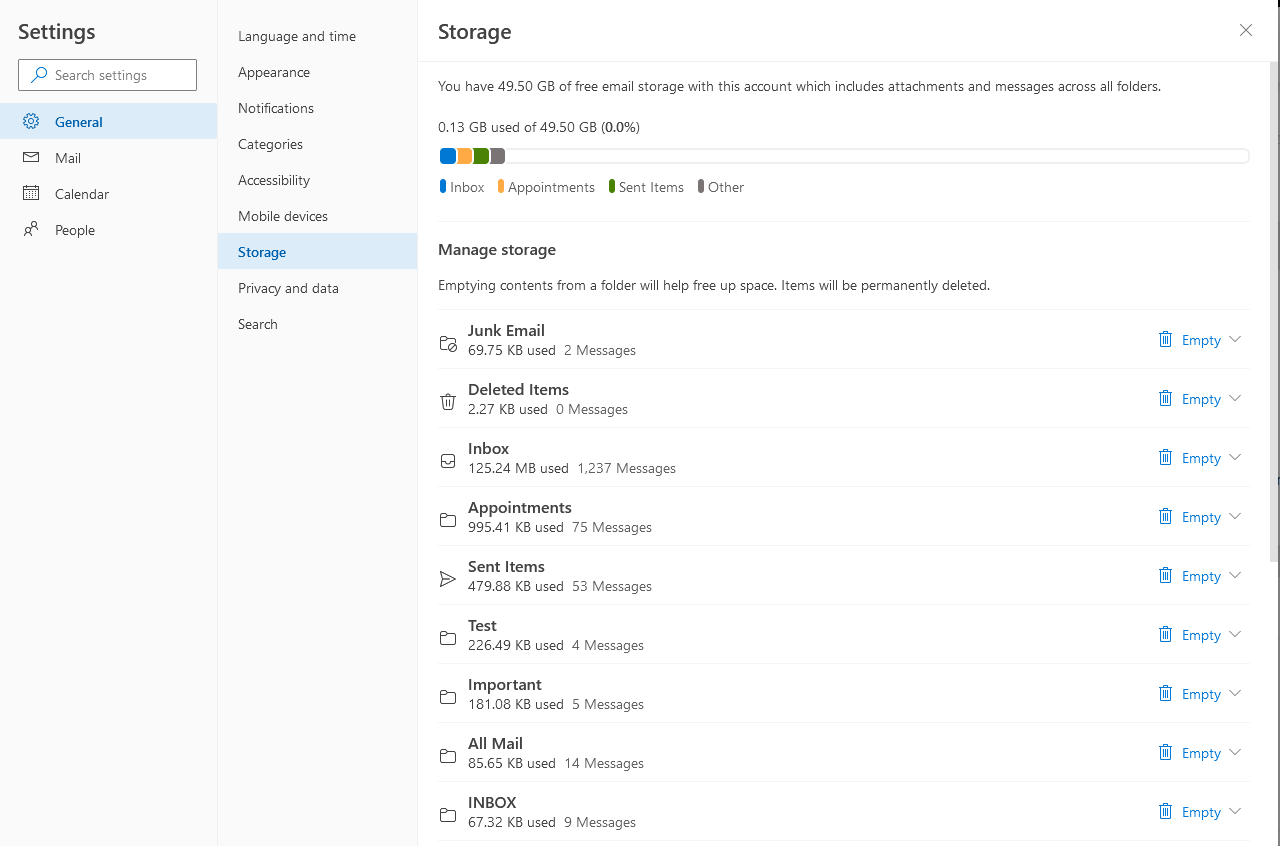**Detailed Caption:**

This image displays a settings menu interface divided into a light gray and white background. The left third features a light gray section, while the remaining area is white, separated by a vertical black line. 

In the top-left corner, bolded in black, is the word "Settings," with a white search bar situated directly underneath it. Below the search bar is a blue rectangle containing a blue settings icon and the word "General" written in blue.

Listed under "General" are three black icons associated with "Mail," "Calendar," and "People." The light gray section continues downward but remains empty until reaching the bottom.

On the right side, still within the light gray background, several options are presented in black lettering: "Language and Time," "Appearance," "Notifications," "Categories," "Accessibility," "Mobile Devices." Another blue rectangle appears, highlighting the word "Storage" in blue. Beneath this are more options in black: "Privacy and Data," and "Search."

Moving to the white background, the top-left corner carries the bolded black title "Storage" with a small "X" on the right side. Below this, a status bar indicates the email storage usage, stating ".13 GB used of 49.5 GBs." A horizontal line spans across the section with segments in blue, yellow, green, and purple, representing different data categories, with white occupying the remainder. Below this line, a legend explains the color codes.

In black text, it states "Manage your storage" with additional instructions noting that "emptying contents for a photo will help free up space." Below this, a vertical list of ten icons appears, each correlating to storage categories such as "Junk Mail," "Deleted Items," and "Inbox."

Each category provides details on the kilobytes used and the number of messages. Adjacent to each category, there is an "Empty" link in blue, paired with a blue trash can icon to its left.